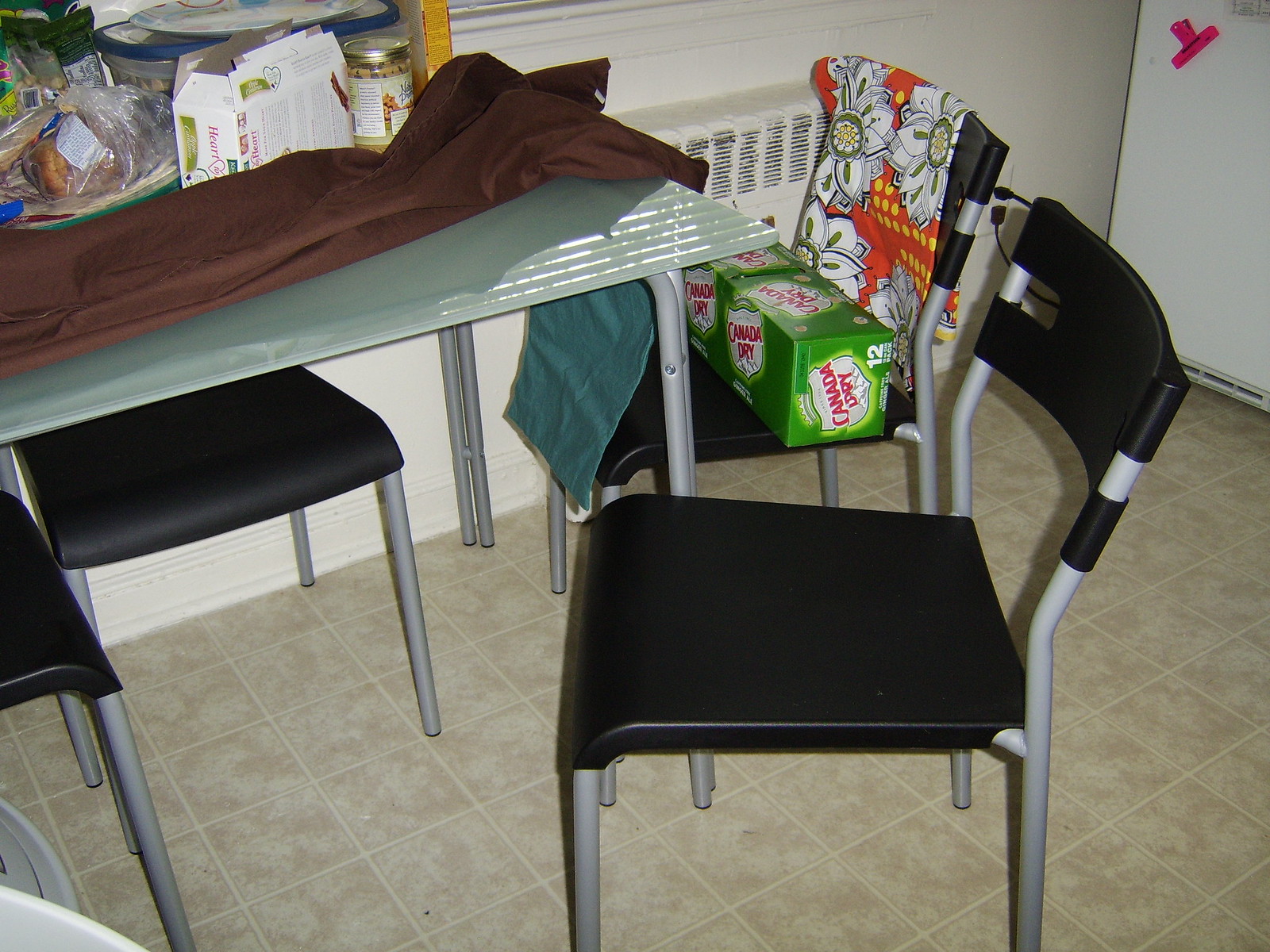In this image, the setting appears to be the interior of a house. Central to the scene is a gray table covered with a brown tablecloth. Spread across the table are various food items. Surrounding the table are four black chairs. The chair on the left has a green box with the "Canada Dry" logo and text, indicating it contains 12 Canada Dry beverages. Draped over the back of this same chair is a cloth featuring a floral pattern in shades of orange and yellow.